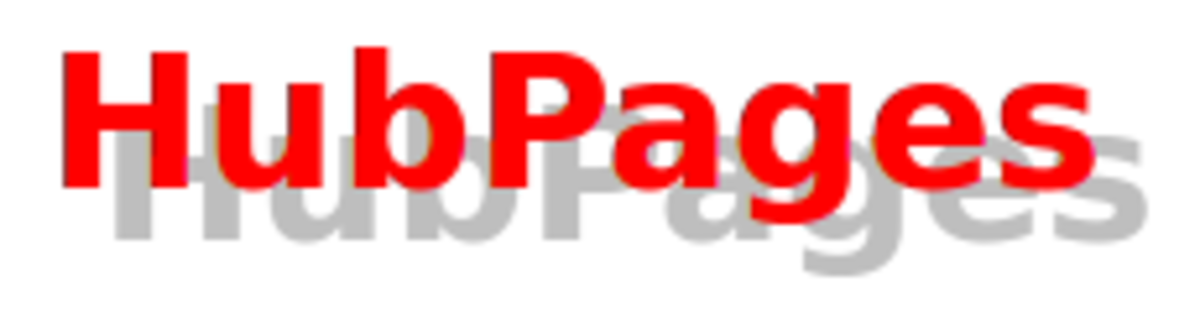In this image, the text "HubPages" is prominently displayed across the top. Each letter is bold and rendered in a vivid red color with a slight bloom effect on the left side, adding a touch of black for depth. The sequence begins in the top left with an uppercase "H," followed by a capital "U," and then a lowercase "b." This pattern continues with a capital "P" positioned towards the top center, followed by an "A," "G," "E," and finally an "S," all in uppercase and consistent in their striking red hue.

The background of the image features a subtle shadow effect, with the word "HubPages" repeated in a light gray color. This secondary text is offset slightly to the right, creating a layered and dynamic appearance. The entire composition is set against a clean, white backdrop, emphasizing the boldness of the main red text while the shadowed gray text adds depth and dimension.